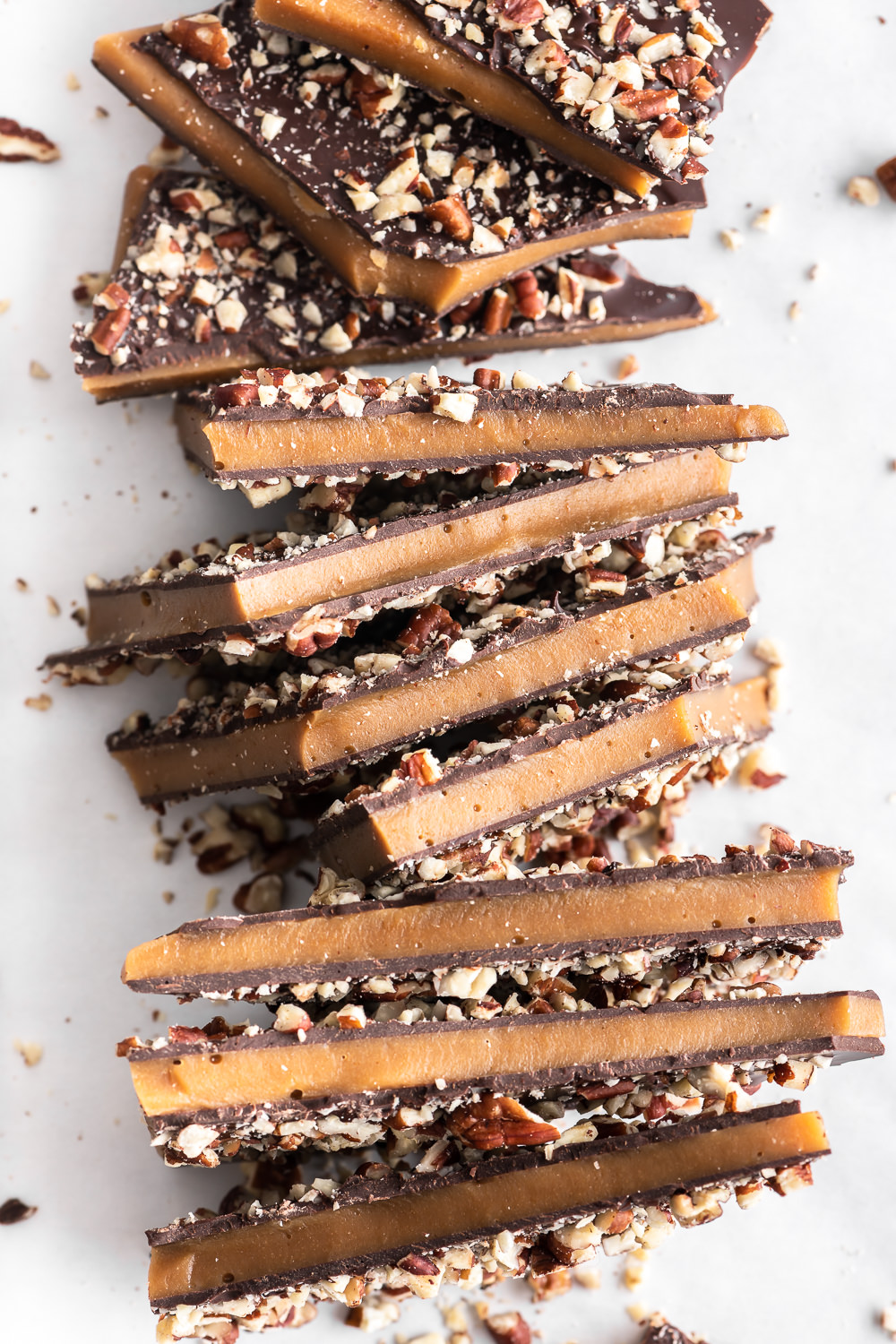This intriguing photograph features approximately ten to twelve thin caramel bars stacked unevenly, much like a tower slightly leaning to the side. The stack is placed on a white tabletop, viewed from an overhead perspective, with the background seamlessly merging with the white surface below. Each bar consists of multiple delectable layers: a base layer resembling a praline crunch or a flat graham cracker-style cookie, followed by a rich layer of caramel. These layers are generously coated in glossy chocolate and topped with crushed nuts, likely pecans. The intricate details of the treat exhibit a tempting combination of crunchy and smooth textures, promising a delightful experience for chocolate and caramel enthusiasts. A few scattered nuts can be seen at the base, adding to the overall visual appeal and hinting at the treat's crunchy consistency.